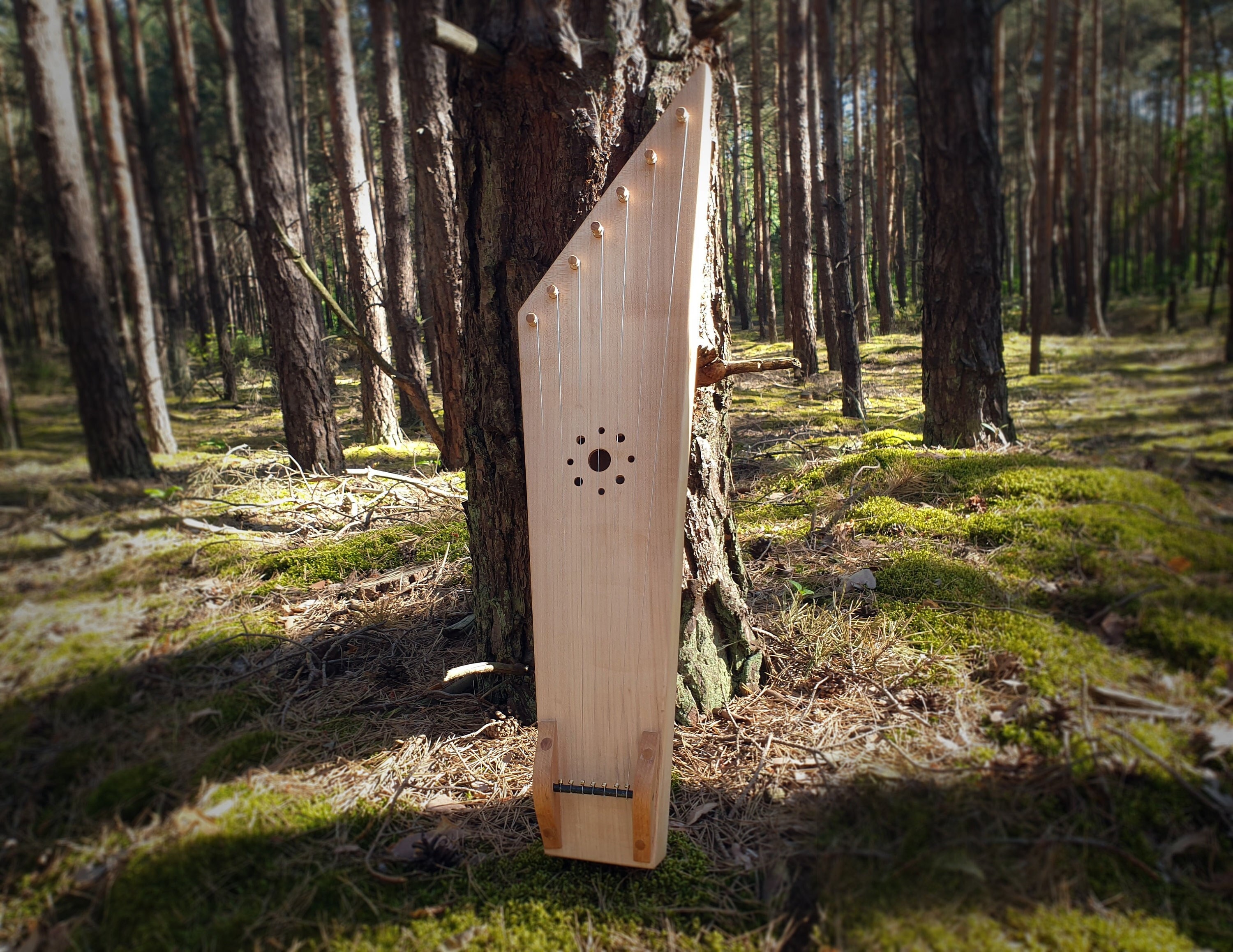In this daytime forest scene, the sun filters through the canopy, illuminating a distinctive homemade stringed instrument prominently placed in the foreground against a backdrop of tree trunks and a lush, moss-covered ground, interspersed with dry patches. The instrument, resembling a hybrid between a guitar and a harp, features a wooden body that narrows at the bottom and widens towards the top, culminating in a diagonal top edge. Centered within its wooden frame is a resonation hole. The instrument is equipped with seven strings, each attached to metallic gold tuning pegs at the top and secured to a small black bar at the bottom, which is adorned with tiny metallic shapes for individual string adjustment. This striking image, with its rustic charm, appears to showcase the craftsmanship and unique design of the instrument, set against the serene and picturesque backdrop of the forest.